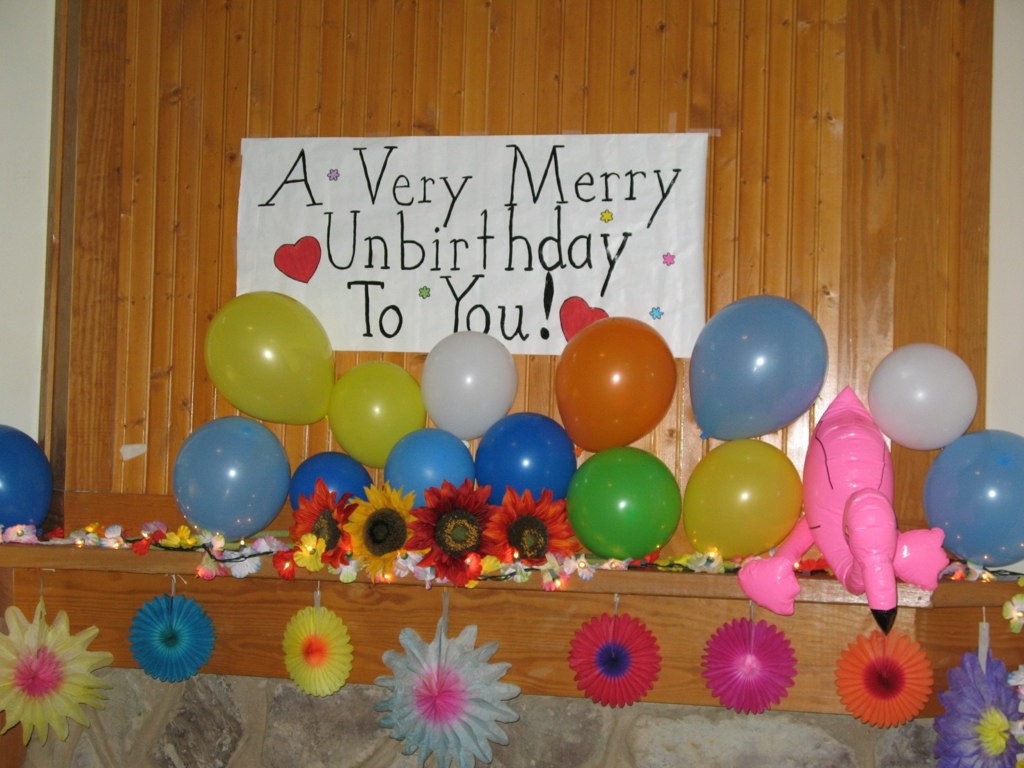The full-color indoor photograph captures a celebratory scene with a distinct retro aesthetic, suggested by the vertical wood plank paneling reminiscent of the 70s or 80s. The focal point is a white sign with black letters that jubilantly exclaims, "A very merry unbirthday to you!" decorated with a red heart and colorful star-like accents. This sign is pinned above a fireplace mantle, which is adorned with festive decorations. 

Atop the wooden mantle are a variety of vibrant paper decorations that resemble sunflowers, crafted in hues of blue, yellow, red, orange, and pink, with different colored centers. These paper flowers fan out gracefully, interspersed with string lights akin to Christmas lights, adding a whimsical touch to the display.

Additionally, a plethora of balloons in assorted colors—yellow, light blue, green, orange, and white—are scattered across the scene, adding to the jubilation. Notably, there is a deflated pink balloon, shaped like a flamingo, lying to the right side of the mantle, contributing a playful and slightly quirky element to the overall setup. The lower part of the image reveals more of the wood paneling, complemented by a section of brick or cement at the bottom, grounding the lively decorations in a cozy, vintage indoor environment.